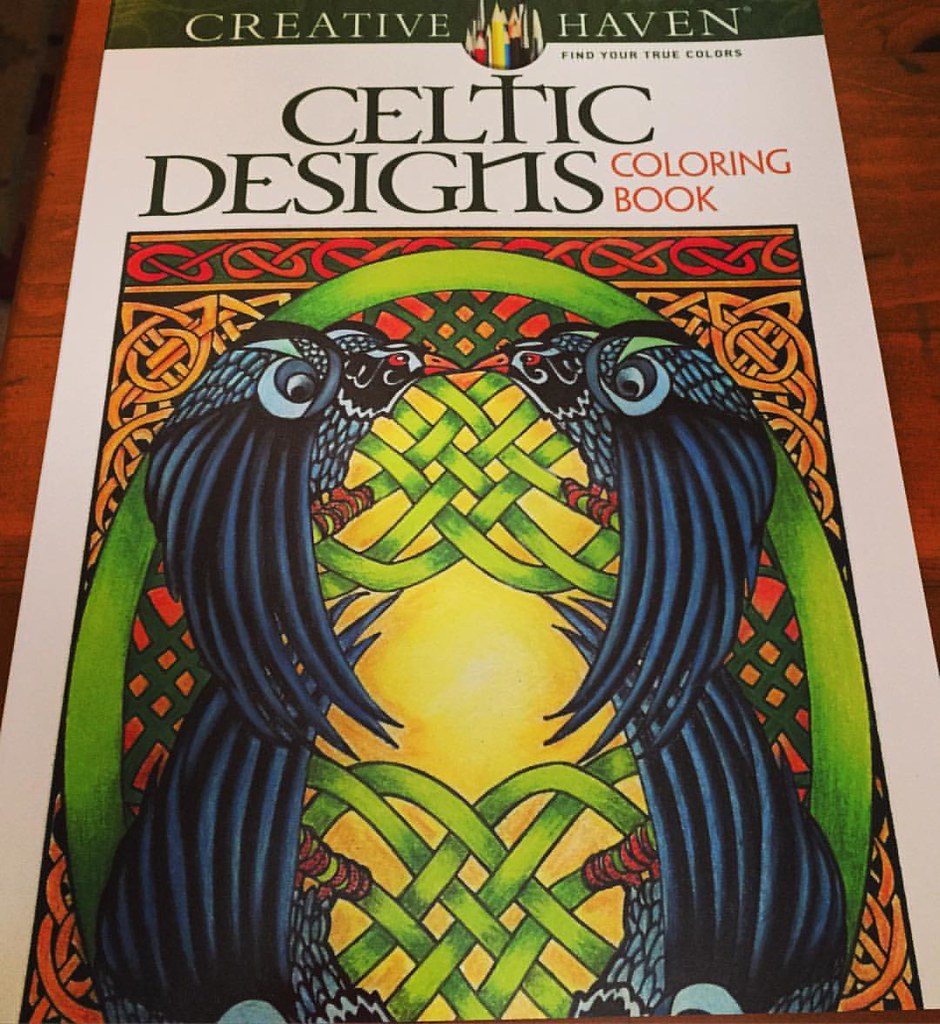In a richly detailed church mosaic, two magnificent birds, resembling black eagles or crows, are depicted upside down, facing each other in an almost symmetrical arrangement. Their plumage exhibits intricate patterns of black and blue, while piercing red eyes and red claws add a striking contrast. The birds are grasping intertwined green ribbons, bringing a sense of fluidity and movement to the piece. The mosaic's background is predominantly red, enhancing the dramatic and almost otherworldly atmosphere of the scene.